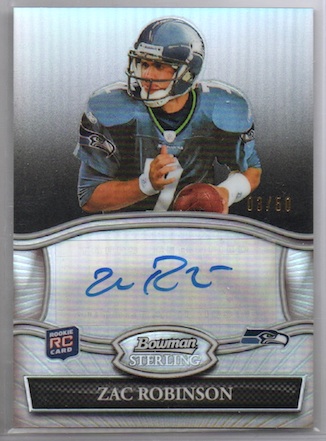This detailed football trading card features a half-body image of Zach Robinson, a player for the Seattle Seahawks, clad in a metallic light blue or greenish-gray jersey and matching shiny helmet. With white sweatbands on both arms, he holds a football in his right hand while looking to his left. The upper part of the card showcases a white-to-black gradient background, adorned with the Seahawks logo on his shoulders. A prominent blue autograph sprawls across a white patterned background in the middle section. The card also boasts a silver border and a special insignia for Bowman Sterling. An embossment near the bottom reveals Robinson's name in silver text on a black carbon fiber-like bar. A gold stamp indicating "03/50" highlights the card's limited production run, making it a rare collector's item.